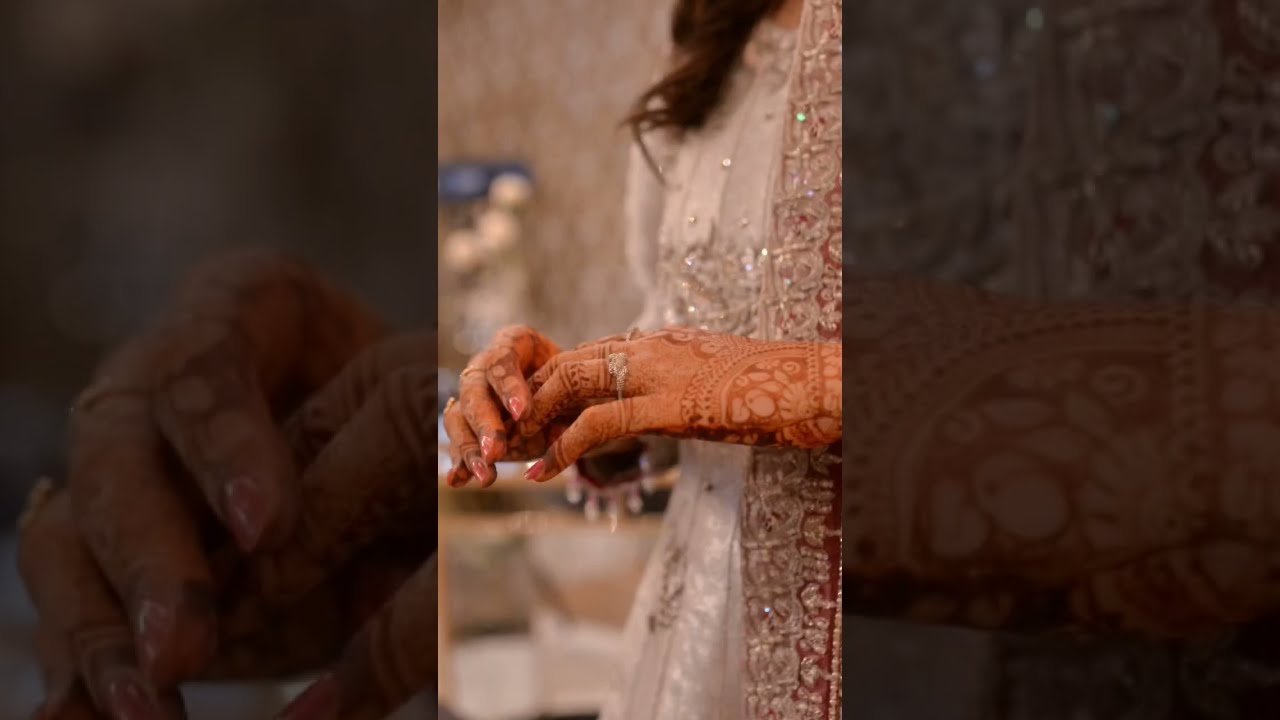The image is a three-panel color photograph prominently featuring a woman adorned for what appears to be a traditional Hindi wedding ceremony. The central panel displays a close-up of the woman's hands, which are elaborately decorated with intricate henna tattoos, also known as India ink tattoos. She wears a ring with small diamonds on her left ring finger, adding a touch of elegance and class. Her attire is a mix of traditionally Indian garb with a white lacy dress that has shiny rhinestones and crystals hanging from it, creating a beautifully intricate pattern that matches the tattoo designs on her hands. Her long brown hair drapes over her right shoulder, cascading down past her shoulders. The background is blurry, but it hints at some sort of display with wallpaper behind her. The left and right panels are close-up, zoomed-in sections of the central image, highlighting the detailed henna tattoos and contributing to the overall intricate and elegant aesthetic of the photograph.